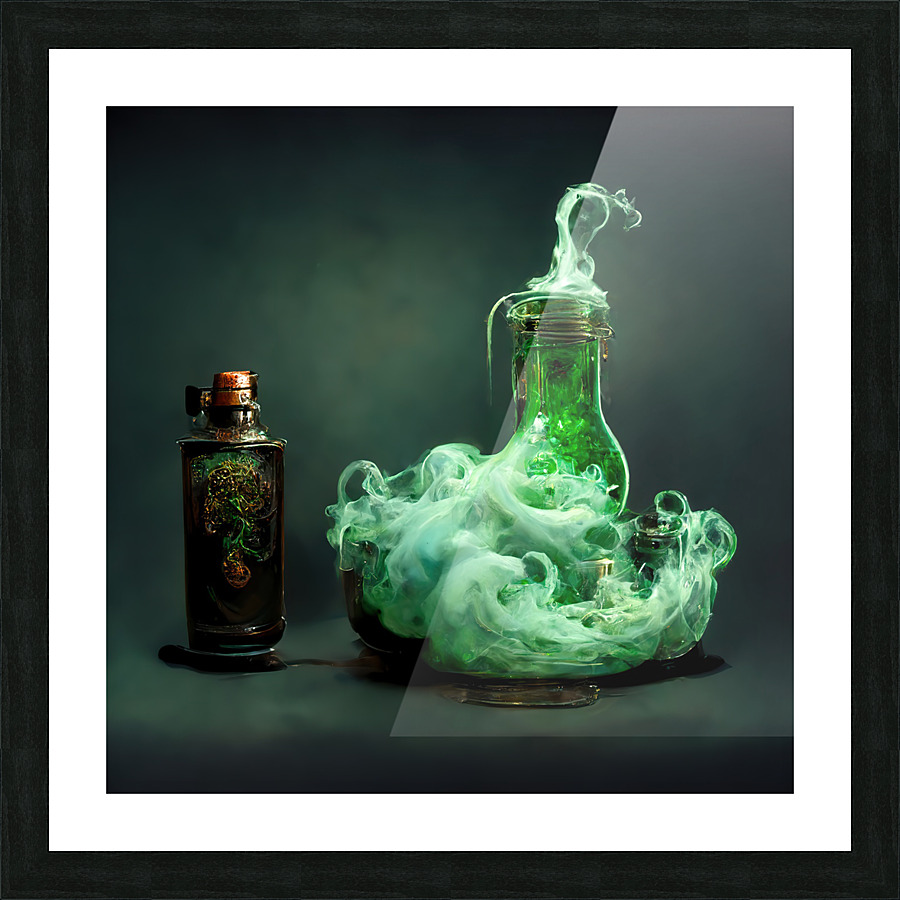The image is a framed piece of artwork featuring two bottles. The frame is black with a white mat surrounding the inner artwork. The background is split diagonally from the top right to the bottom left, with a dark green backdrop on the left side and a light gray backdrop on the right. 

On the right side of the image, there is a glass jar or beaker filled with neon green liquid. Wispy green smoke emanates from the top, enveloping the jar and spreading across the bottom and surrounding area. Upon closer inspection, silver stems can be seen protruding from both sides of this jar.

To the left of the glass jar, there is a dark-colored bottle adorned with a vibrant, multicolored pattern resembling a tree or growth, featuring shades of green, yellow, and red. The bottle is capped with what appears to be a red lid. Between the two objects, some liquid seems to have spilled.

Overall, the artwork sharply contrasts the vividly detailed bottles against the dual-colored background, combining elements of scientific imagery and decorative design.